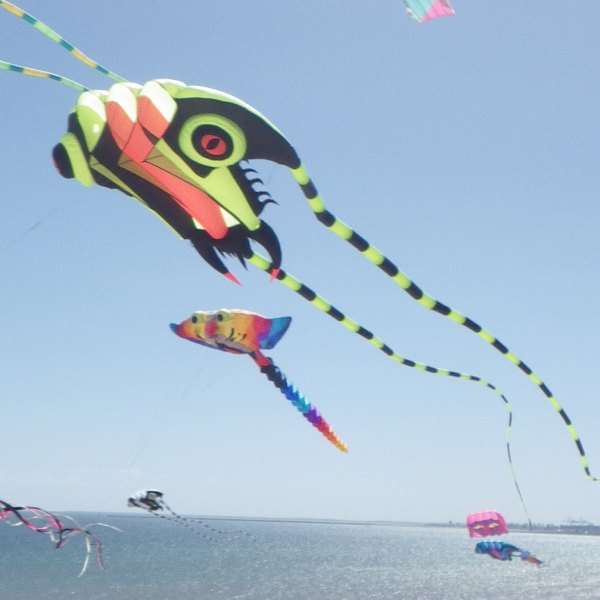This outdoor photograph captures a vibrant display of kites soaring over a large body of water, likely the sea, with a clear blue sky as the backdrop. The water below shimmers with sunlight, providing a gleaming canvas. The kites are intricately designed and magnificently colored, each adorned with long, flowing tails. The kite closest to the camera resembles an alien bug with two long, light green and black striped tails, green and blue antennae, a black and green body, and a striking red eye. Below it and further back, a kite shaped like a stingray or manta ray has a multicolored tail featuring shades of blue, purple, and orange, and two large eyes on its front. Additional kites in the distance boast equally vibrant designs, such as one with a rainbow-colored tail and another featuring yellow and black alternating stripes. A city is faintly visible along the shoreline in the distance, adding a subtle urban touch to this otherwise natural and whimsical scene.